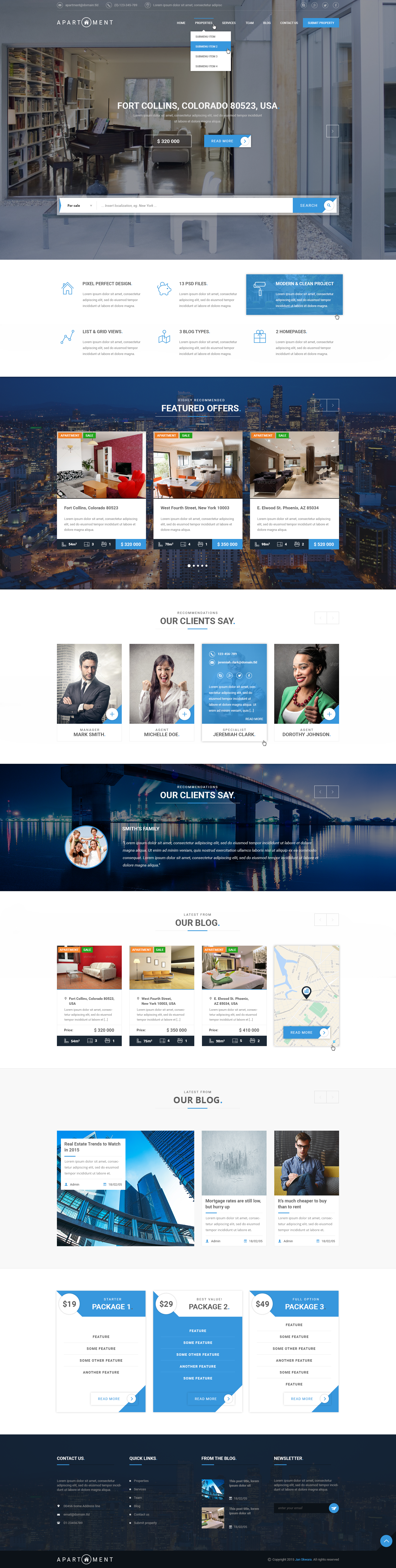### Detailed Descriptive Caption for Real Estate Image in Fort Collins, Colorado

This image showcases a cutting-edge real estate property listing platform, focusing primarily on Fort Collins, Colorado. The interface highlighted here is designed to ease apartment searches, featuring pixel-perfect design, list and grid views, and includes 13 PSD files with three blog types. The platform boasts a modern and clean aesthetic, offering two homepage variations to cater to different user preferences. 

The system underlines several featured property offers. Detailed information about the search results includes properties in Fort Collins with a remarkably small and crowded apartment priced at $320,000, potentially due to excessive furniture. This property includes a fireplace and is situated on West 4th Street in New York, where a more spacious apartment is listed for $350,000. Additionally, a high-value penthouse in Phoenix, Arizona, is shown with a price tag of $520,000, although it is irrelevant to the initial Fort Collins search criteria.

Further insights introduce key personnel associated with the listings. The team comprises Mark Smith, the manager, who is seen wearing a suit and tie; Michelle Doe, an agent, dressed in a button-down shirt with long hair; Jeremy Clark, a specialist; and Dorothy Johnson, wearing a green blazer with a tank top.

The platform also includes a map feature to highlight property locations and a detailed breakdown of real estate market trends of 2015, albeit in a foreign language. These trends emphasize that mortgage rates are low, making buying more affordable than renting. 

For those interested in listing properties, the platform offers three package options:
1. **Starter Package** - $19: Includes basic features.
2. **Best Value Package** - $29: Contains several enhanced features.
3. **Full Option Package** - $49: Provides a comprehensive suite of features.

Lastly, the interface integrates a ‘Contact Us’ section, quick links to blog posts, and a newsletter signup, with some of the information displayed in foreign languages.